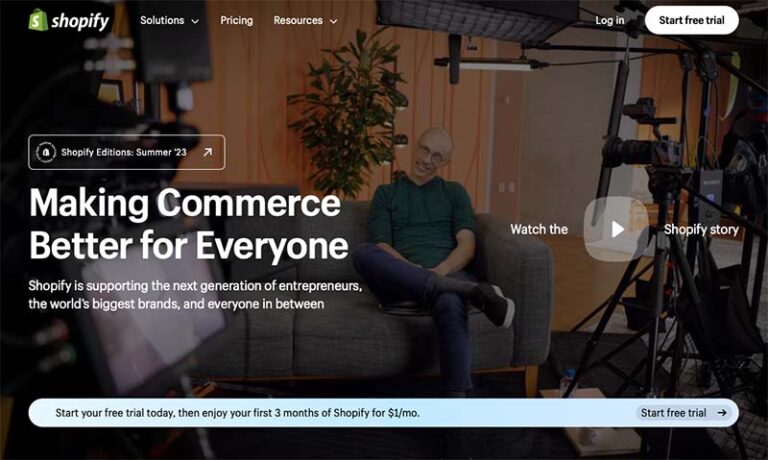This is a detailed caption for the described image:

In the screenshot of the Shopify website, the top left corner features a green shopping bag icon with a white "S" in it, followed by the "Shopify" name. The navigation bar across the top includes three menu items: "Solutions" with a drop-down menu, "Pricing," and "Resources" with a drop-down menu. On the right side of the navigation bar, there is "Log In" in white text and a prominent white button with black text that reads "Start Free Trial." 

The background has a dark overlay that partially obscures an image of a person sitting on a couch surrounded by video equipment. On the left side, a white-bordered box contains text that reads "Shopify Edition Summer '23" with an upward and rightward pointing arrow. Below this box, a large title states, "Making commerce better for everyone," followed by body text that explains, "Shopify is supporting the next generation of entrepreneurs, the world's biggest brands, and everyone in between." 

To the right of this text, there is a call-to-action that says, "Watch the Shopify story," with a semi-transparent white play button situated between "the" and "Shopify." 

At the bottom of the page, there is a gradient banner transitioning from white to blue, containing the text, "Start your free trial today then enjoy your first three months of Shopify for $1 a month." Within this banner, there is another button with the text "Start Free Trial" accompanied by an arrow pointing to the right.